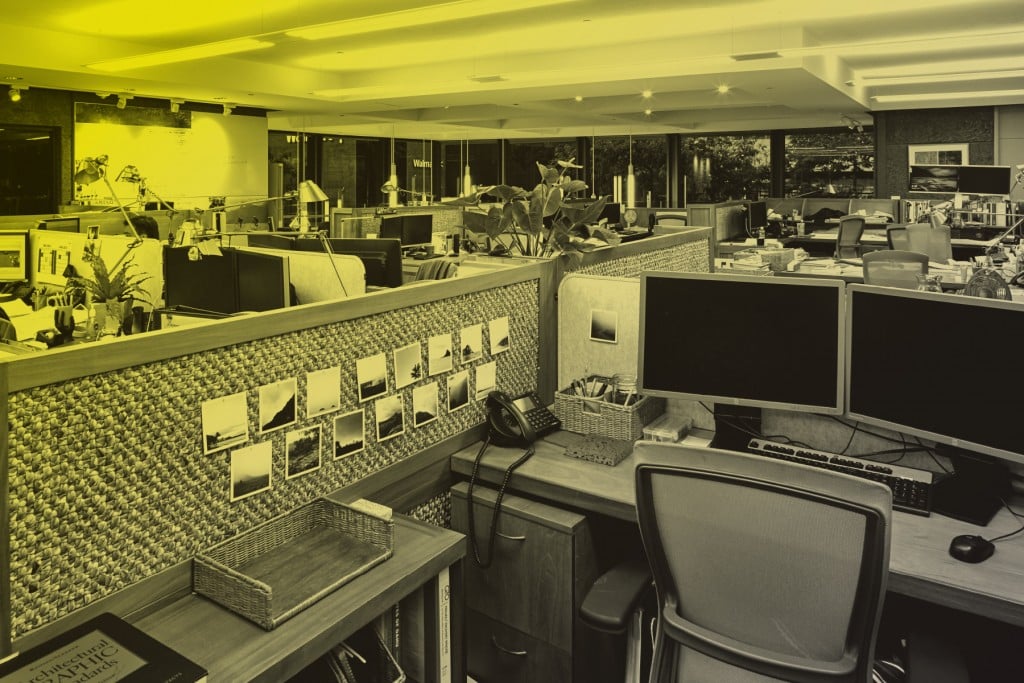The image depicts the interior of a shared office workspace, featuring a series of cubicles divided by partitions. In the immediate foreground, one cubicle is prominently visible, furnished with a chair and a desk that houses two desktop monitors connected to a CPU, along with a keyboard and mouse. The desk is also adorned with a wicker basket, a landline telephone, and various accessories such as pencils. Photographs are affixed to the cubicle wall on the left side, adding a personal touch to the workspace. To the left of the main cubicle, there are trays for organizing documents. Additionally, neighboring workstations are enhanced with potted plants. Overhead, the ceiling is fitted with lights that illuminate the office space. The overall color scheme of the image is a distinctive black and white with a greenish tint, adding a unique stylistic quality to the scene. In the distance, a man is visible working in one of the cubicles, with a lamp situated in front of him and a drawer beneath his desk.